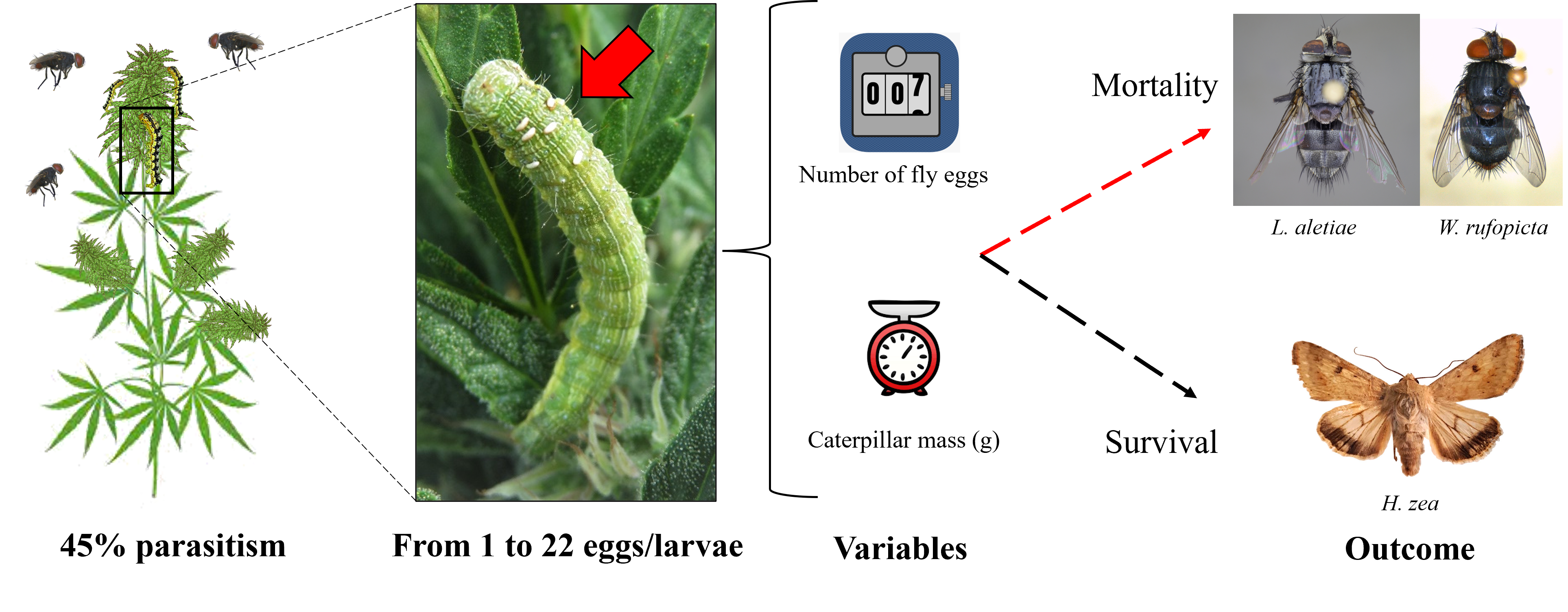The image is an informational graphic focusing on parasitism in caterpillars. On the left side, the graphic indicates "45% parasitism" and features a caterpillar situated on a leafy plant, speculated to be a marijuana or sativa plant. The caterpillar is emphasized within a black rectangle, and nearby, two other caterpillars are visible among the leaves, with flies hovering above.

To the right, a blown-up image of the caterpillar shows white eggs or larvae on its back, specified as "from 1 to 22 eggs/larvae". The graphic uses a red arrow to point to these white blobs. Further right, there's a section labeled "number of fly eggs" with a counter going up to seven, and another labeled "caterpillar mass in grams". These are listed under the category "variables".

Two arrows stem from these variables: the top arrow points to "mortality" and features images of two flies, LLTA and W. aruthopicta, while the bottom arrow points to "survival" and depicts a moth, indicating the "HZ outcome".